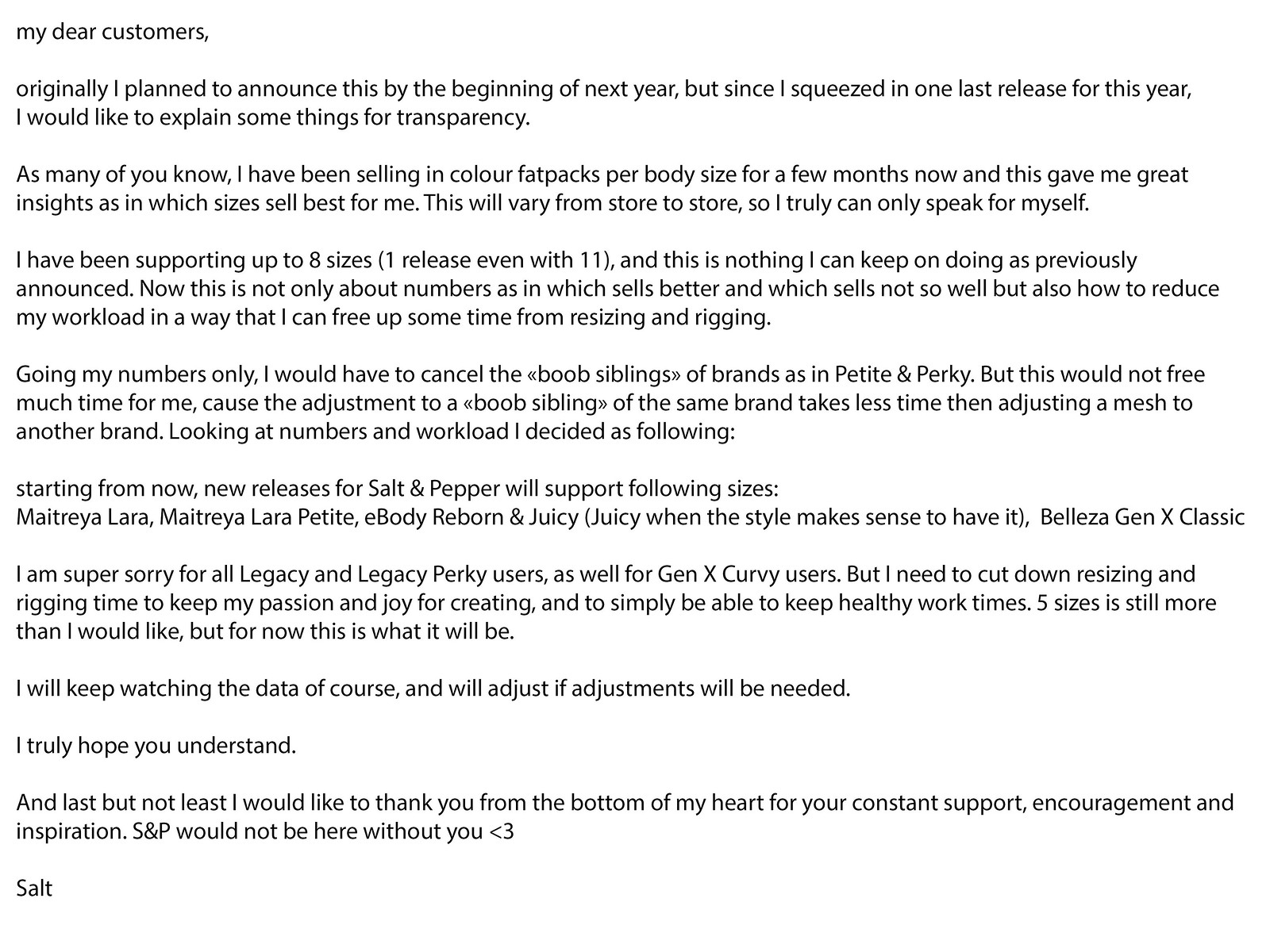The image depicts a detailed letter or email addressed to customers from a seller named Salt. The letter begins with “My Dear Customers” and explains that an announcement initially planned for the beginning of next year is being communicated earlier due to an additional release for this year. Salt has been selling color fat packs per body size for a few months, which provided insights into the best-selling sizes. The seller has been supporting up to eight sizes, with one release including eleven, but has decided to reduce this number to manage workload and maintain a passion for creating.

The core issue discussed is the need to cut down on resizing and rigging time, not solely based on sales numbers, but also to free up time for healthier work practices. Despite the data suggesting a need to possibly cancel certain sizes, like the Petite and Perky adjustments, Salt explains these do not significantly impact workload compared to other tasks. 

From now on, new releases for Salt and Pepper will support the following sizes: Matriolara, Matriolara Petite, eBody Reborn, Juicy (when stylistically appropriate), and Bezella Gen X Classic. Unfortunately, support for Legacy, Legacy perk, and Gen X curvy users will be discontinued to streamline workflow. Although this still means supporting five sizes, it's a necessary step.

Salt concludes the letter with heartfelt gratitude for the customers' constant support, encouragement, and inspiration, signing off with the name Salt.